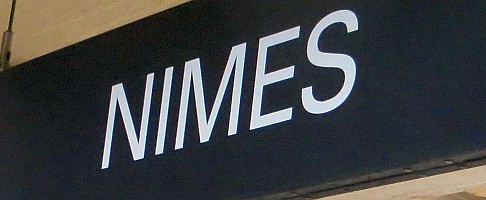The photo depicts a close-up of the top part of a storefront or a building sign. Central to the image is a black board with large, bold white letters spelling out "NIMES" (N-I-M-E-S). The sign appears to be constructed of an indeterminable material, possibly wood or a similar substance. Surrounding the sign and visible in the upper left corner and below the sign is a light brown or beige material that resembles wood or plaster, indicating the building's exterior. A vertical dark line is also visible in the image, which could be grouting or part of the building's structure. Additionally, there seems to be a pole or a structural support on the left side, suggesting this sign might be hanging at the entrance or elevated as a billboard.